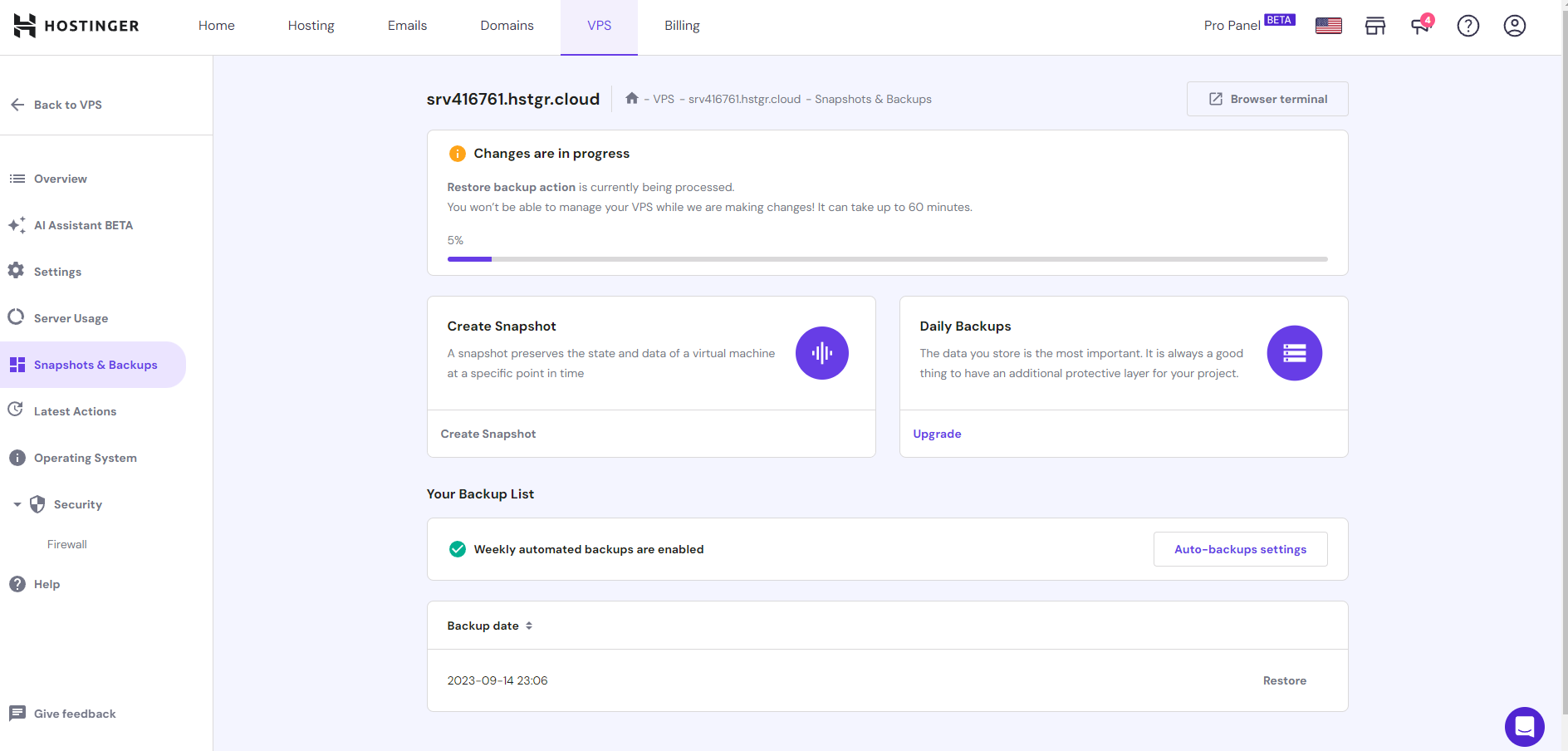In this detailed image, we observe a web application interface, likely belonging to a company named Hostinger, as indicated by its logo and name displayed prominently in the upper left corner. The top navigation bar contains several sections labeled: Home, Hosting, Emails, Domains, VPS (which is highlighted in purple), and Billing. 

To the right of the navigation bar, icons are visible, including an American flag and a user profile icon. Below this bar, the interface divides into a left and main pane. The left pane, colored white, features various navigation buttons: "Back to VPS", "Overview", "AI Assistant", "Data Section", "Setting Section", "Server Usage Section", "Snapshots and Backups" (highlighted in purple), "Latest Actions", "Operating System", "Security", "Firewall", and "Help". At the bottom, there's a "Give Feedback" option.

Dominating the main page, which appears to be the "Snapshots and Backups" section, there's an active progress indicator stating "Charges are in Progress," with a restore action being processed and a visible progress bar at 5%. Further options on this page include buttons for "Create Snapshot," "Daily Backups," and settings for managing backups: "Your Backup List," "Auto Backup Settings," "Backup Date," and "Restore."

Additionally, a distinct purple chat button is positioned in the lower-right corner, offering immediate customer support. The overall design primarily utilizes a light purple background, complemented by white text sections containing relevant information and interactive elements.